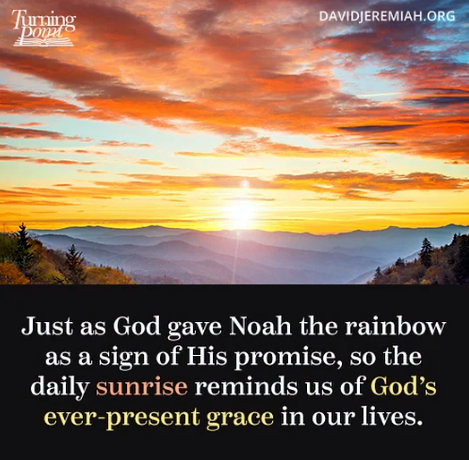This computer-generated image, designed as a Christian-themed poster, showcases a breathtaking sunset in vivid detail. Dominating the top two-thirds of the rectangular poster is a serene sunset scene featuring a gradation of rich hues: shades of blue, orange, red, and yellow. In the background, majestic mountains fade into the distance, and lush greenery frames the landscape on both sides. 

White text in the upper left corner reads "Turning Point," while the upper right corner displays "DavidJeremiah.org" in capital letters. The bottom third of the image is a black band with a powerful inspirational quote rendered primarily in white text. The key words within the quote are highlighted in different colors for emphasis: "sunrise" appears in orange and "God's ever-present grace" in yellow. The full quote reads, "Just as God gave Noah the rainbow as a sign of His promise, so the daily sunrise reminds us of God's ever-present grace in our lives," encapsulating a message of hope and divine presence.